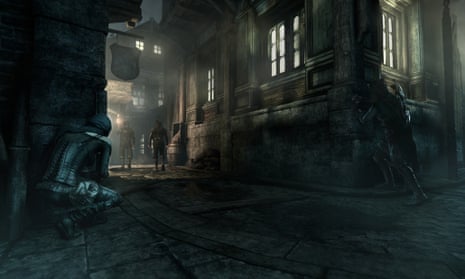This color, landscape-format image appears to be a computer-generated scene reminiscent of a video game, depicting a tense nighttime scenario set in the Middle Ages. The perspective is from a low, crouched position on a cobblestone street in an outdoor village or town. The scene shows two men hiding behind corners of stone buildings on opposite sides of the street, each intently watching two figures—potentially guards or other men—approaching in the distance. The mood is stealthy and foreboding, enhanced by the darkness and the faint glow from what might be candlelight in the windows, suggesting a late-night ambush or a planned attack. The exact attire of the men is difficult to discern, though it possibly resembles armor, adding to the medieval ambiance.